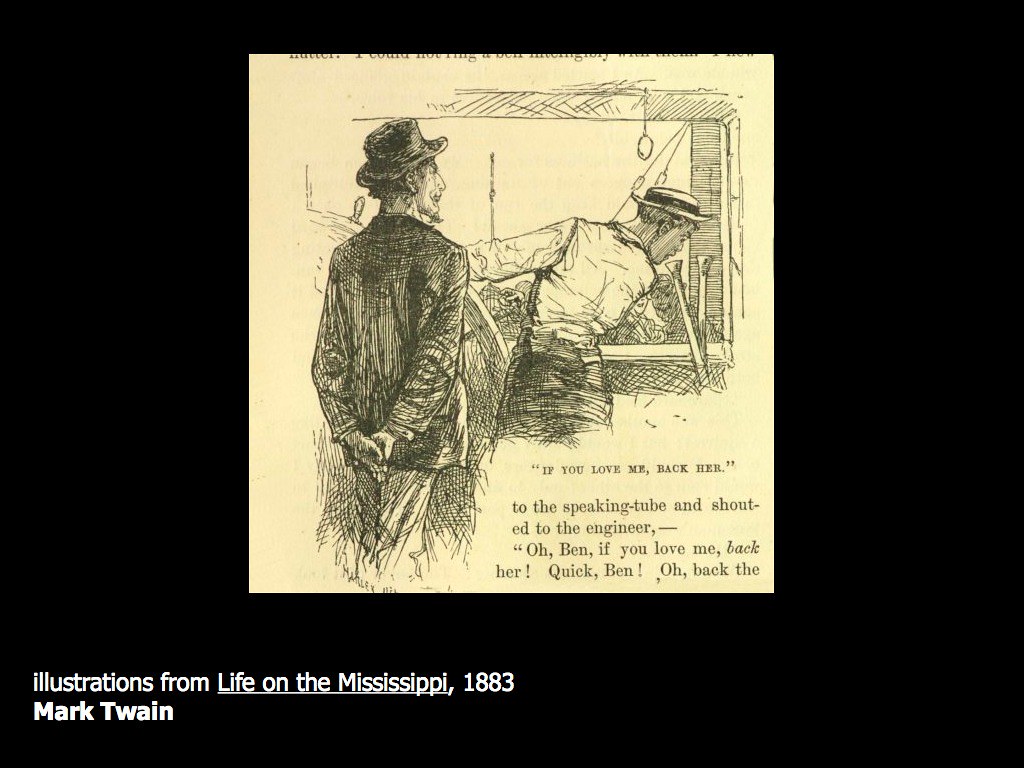The image is a historical sketch with a black background and a text at the bottom in white, reading "Illustrations from Life on the Mississippi, 1883, Mark Twain." The blackness forms an uneven border around this page, accentuating the sepia-toned drawing that seems to have aged over time. The sketch depicts two men from behind. The man in the foreground wears a black suit coat and a tall, black-brimmed hat. His arms are clasped behind him as he gazes off to the right. In the background, another man is visible, steering a ship. He dons a white brimmed hat and a white shirt, looking down towards the bottom right corner. In this corner, an excerpt from the book reads, "If you love me, back her to the speaking tube and shouted to the engineer, oh Ben, if you love me, back her. Quick, Ben, oh back the..." Shadows swallow the rest of the scene, highlighting the historical and nautical ambiance of the setting.